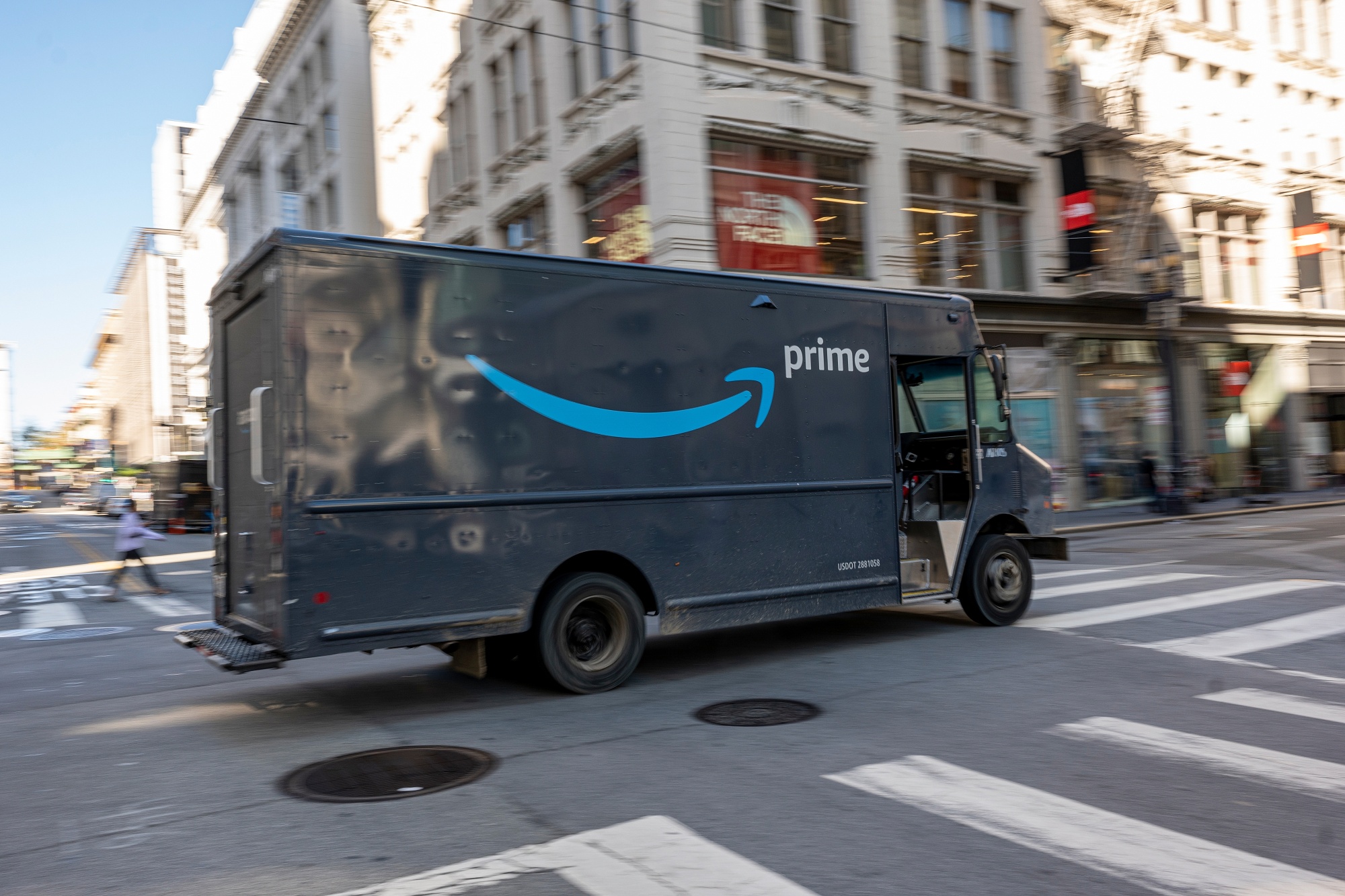A dark navy blue Amazon Prime delivery truck is prominently featured in the image as it drives along the road. The truck is adorned with a distinctive light blue curved arrow that extends from the left side, curving up to the right and pointing towards the word "prime," which is boldly written in lowercase white letters: "prime." One of the truck's delivery doors on the right side is open, revealing two silver steps for entering and exiting the vehicle.

In the background, a cluster of tall buildings looms, including a storefront for The North Face. The store's facade is identified by a red square in the window, with "The North Face" inscribed in white text accompanied by white lines to its right.

Adding life to the scene, a person is seen walking in the background, crossing the street behind the Prime truck. In the bottom right corner, noticeable white lines mark the pedestrian crosswalk, indicating a safe passageway for pedestrians. The Amazon Prime truck appears poised to cross the walkway, integrating the bustling urban landscape and its dynamic movement.